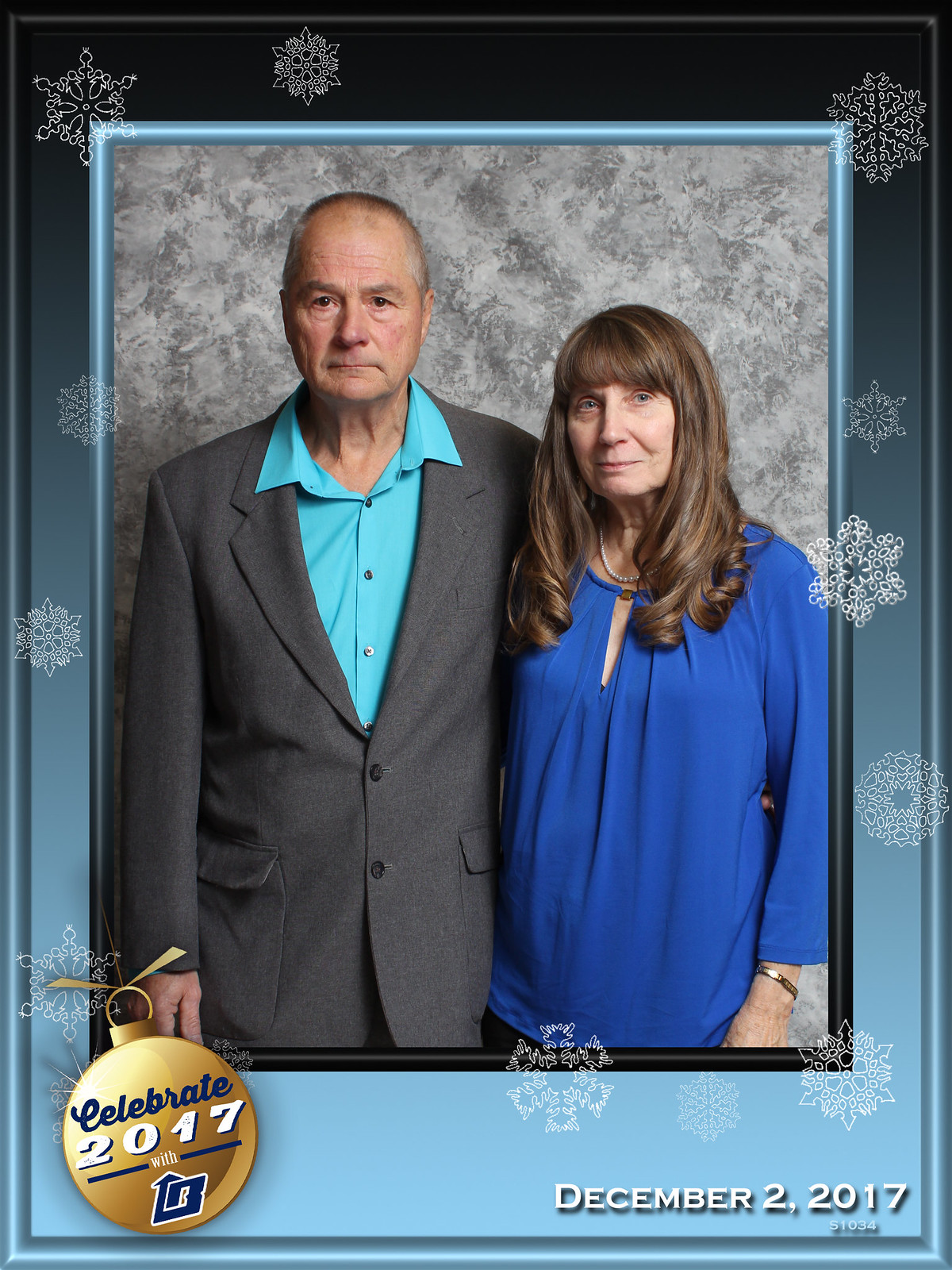This is a digital photograph of a man and a woman framed within a gray border adorned with white snowflakes and featuring a gold Christmas ornament. The text within the image reads "Celebrate 2017" and "December 2nd, 2017". The couple is standing in front of a marble background. The man, who is balding, is dressed in an aqua open-collared shirt paired with a gray sports jacket and has a neutral expression on his face. The woman has long, light brown hair and is wearing a royal blue long-sleeve shirt with a pearl necklace, and she has a slight smile. The man is standing close to the woman with his arm around her back, while both gaze directly at the camera.